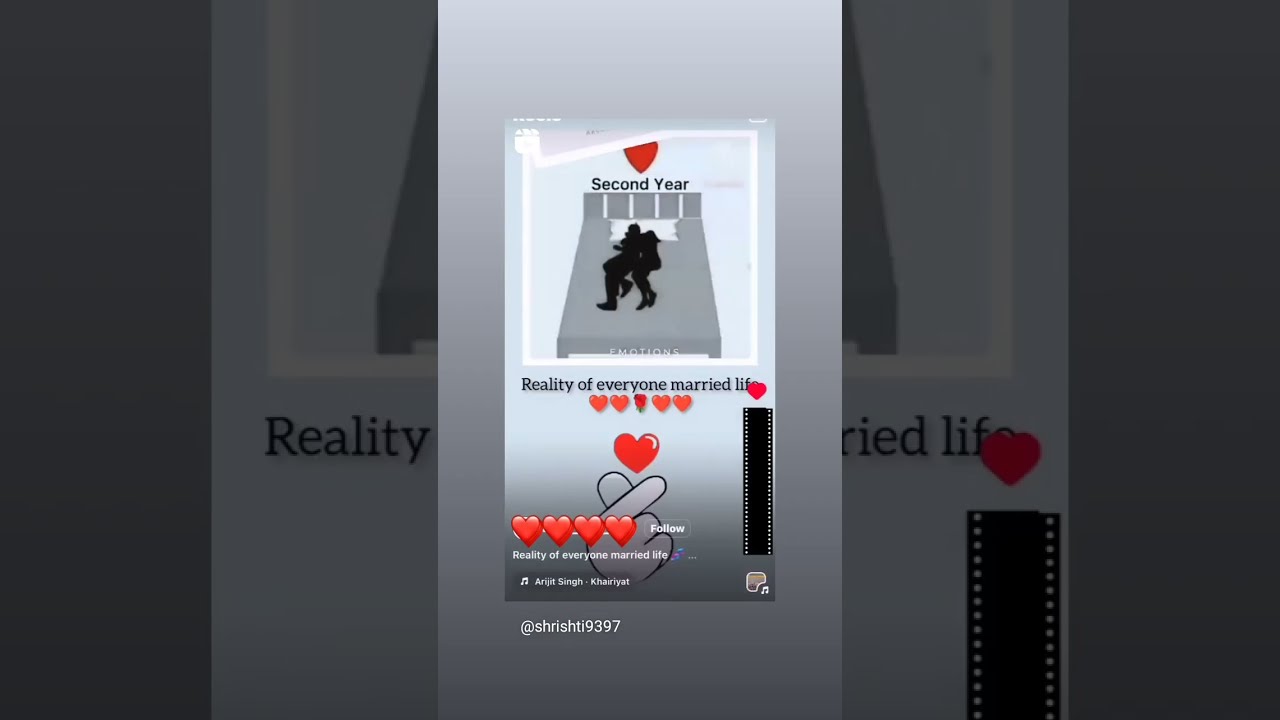The image central panel features a digitally created scene with a grey bed and two completely black silhouettes of people lying side by side, facing left. Above the heads of the silhouettes where the pillows would be, black text reads "second year" and is topped by a red heart with a white border. Below the bed, the phrase "reality of everyone married life" is written in black, followed by a red heart. Further down, there is a sequence of decorative elements, including two smaller red hearts, a rose, and two more red hearts aligned horizontally. Below these elements is a larger red heart and an illustrated hand with the thumb pointing left and the index finger pointing up to the right. Under this hand, there are four additional red hearts next to the word "follow" and a repetition of the text "reality of everyone married life." The background of the main panel is grey, bordered by vertical grey strips on both sides that contain zoomed-in sections of the main image. The left strip zooms in on the word "reality" directly under the bed, and the right strip highlights the heart at the end of the phrase "married life." Additionally, there is a musical symbol followed by a foreign name and an '@' sign with another name at the bottom of the image.